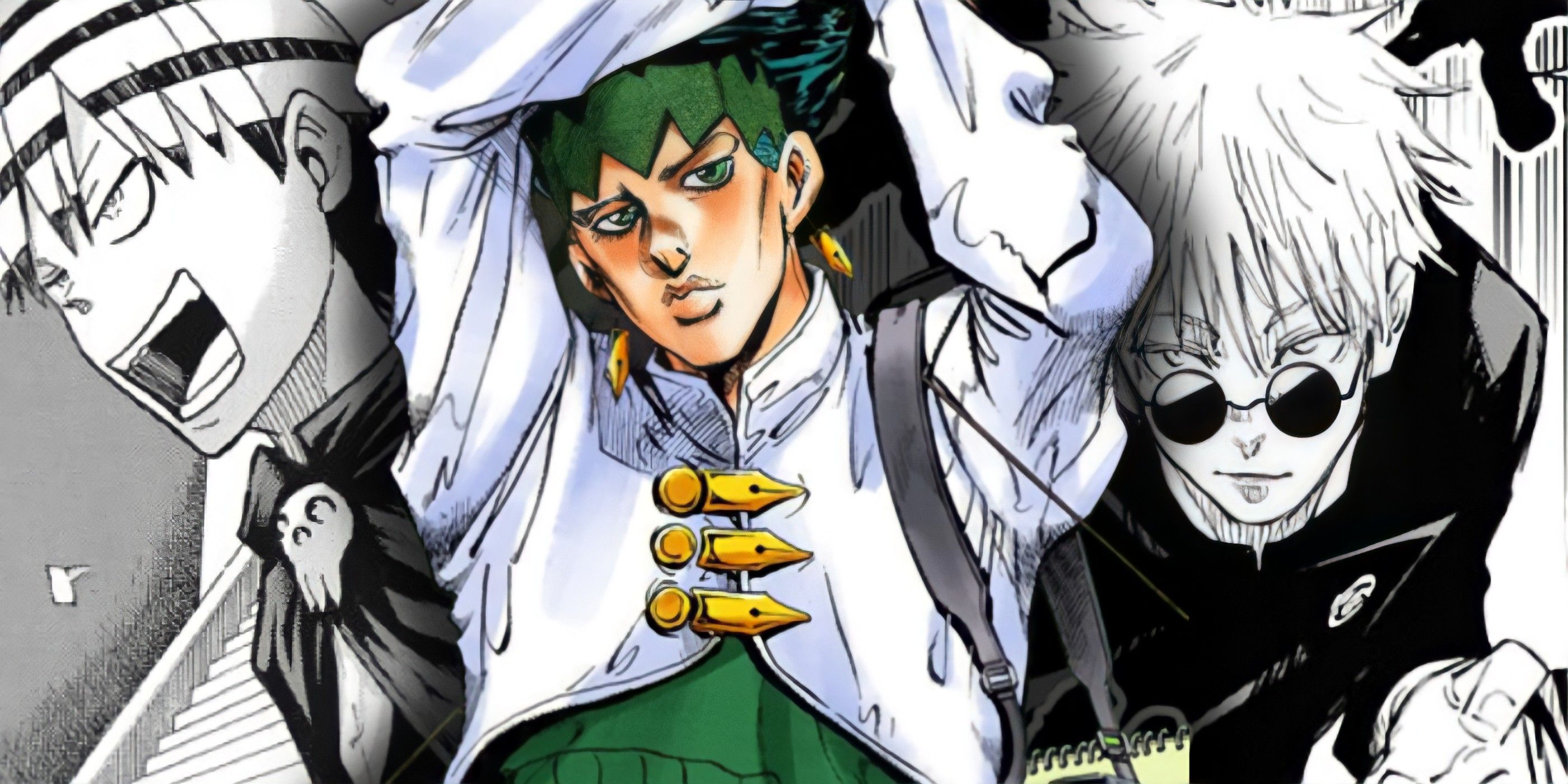This image, reminiscent of a manga or anime page, features three distinct characters. On the left, rendered in black and white, is an animated man with spiky white hair accented by black horizontal stripes. He is shown yelling forcefully, with his mouth wide open revealing his teeth and tongue. He wears a black cape fastened by a skull brooch at the neckline and a scarf around his neck. Behind him, the edge of a steep staircase is visible.

In the center, a vividly colored young man is depicted, standing with his arms raised above his head and his head tilted towards his right shoulder. He has dark green hair, green eyes framed by eyeliner, and a sallow face with high cheekbones. He wears a short, loose-fitting white bolero-style jacket with three gold fasteners resembling pen nibs, over a green shirt that matches the color of his hair. His accessories include gold earrings and what appears to be a holster or bag strap over his left shoulder.

On the right side, another black-and-white character peers out. He has spiky white hair and is wearing dark, round sunglasses. Dressed in a black jacket that features a white logo over the left breast pocket, he stands hunched slightly forward, looking toward the camera. The overall composition suggests that these characters are part of a larger manga or anime series, likely from a narrative with dramatic and dynamic elements.